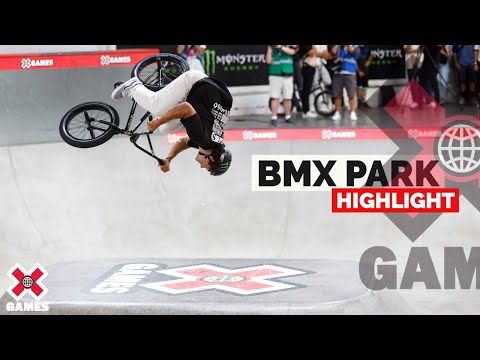In this poster image, a man is performing an aerial stunt on his black bicycle, which is currently upside down, showcasing his skills mid-flip. He is dressed in a black t-shirt, white pants, and grey sneakers, and wears a black helmet for safety. The background features a sleek, gray, and somewhat shiny flat ground, with the X Games logo prominently displayed on it. Crowds of spectators are visible at the front and top right corner of the image, intently watching the performance. On the right side of the poster, semi-transparent text reads "BMX Park Highlight" with "BMX" in black and "Highlight" in white on a red strip. The partially visible X Games logo also appears at the bottom left corner. Additionally, the top and bottom of the poster are bordered by black horizontal strips.